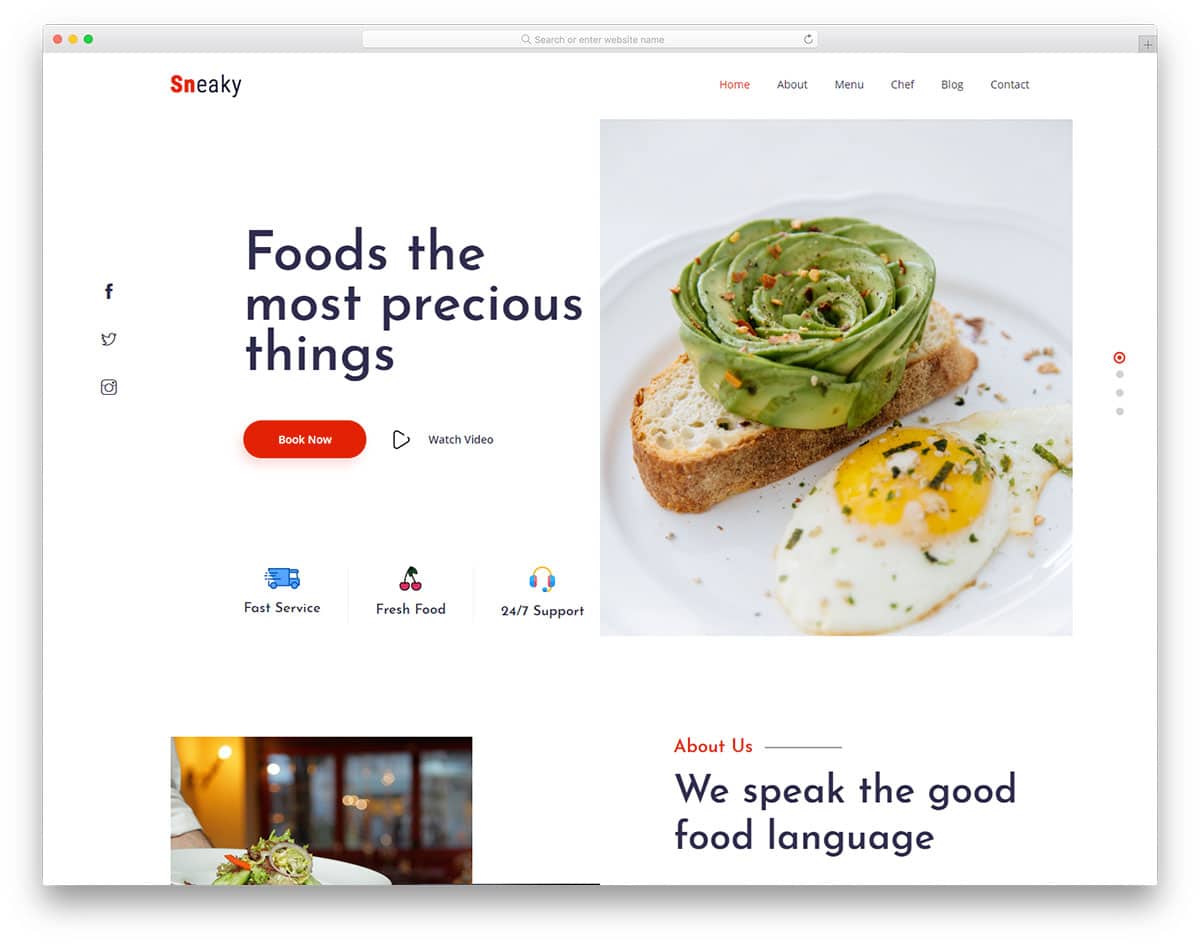This is a screenshot of a website layout. At the top, there is a prominent search bar with the placeholder text "Search or enter website name." On the top left corner, the website's name, "sneaky," is showcased with the "S" and "N" in red, while the remaining letters "E-A-K-Y" are in black. 

To the right, a navigation menu features options including: Home (which is currently selected), About, Menu, Chef, Blog, and Contact. A tagline reads, "Food's the most precious thing," which is grammatically incorrect and should read "Food is the most precious thing."

Below this tagline, buttons for "Book Now" and "Watch Video" are displayed. The central focus is a photograph of a gourmet avocado toast. The dish features a small, crusty slice of baguette topped with sliced avocado arranged in a floral pattern. Accompanying the toast is a perfectly fried egg, with its yellow yolk and crispy edges clearly visible, sprinkled with green herbs. The avocado is dusted with a small reddish-brown spice or powder.

Under the photograph, a text section highlights "Fast Service, Fresh Food, 24-7 Support." At the bottom right of the screenshot, a partial image depicts a person holding a white plate filled with salad. To the right of this image, a section titled "About Us" reads, "We speak the good food language."